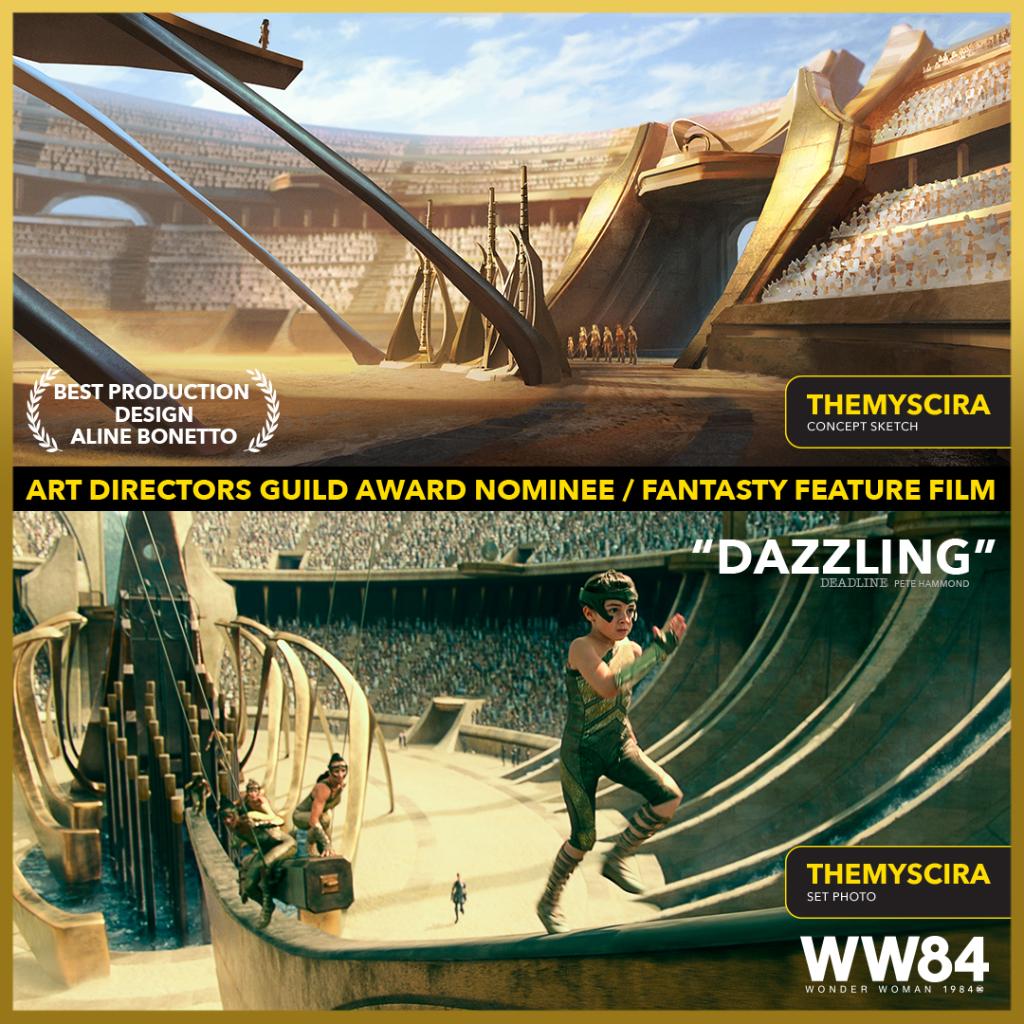This poster features two distinct visuals from the *Wonder Woman 1984* movie. The top half presents a wide-angle concept sketch of the Themyscira stadium, which is reminiscent of ancient coliseums, complete with gold accents and spectators in the stands. Within this top section, a badge on the bottom left corner reads, "Best Production Design, Aline Bonetto," while the bottom right corner is labeled, “Themyscira Concept Sketch.”

The lower half of the poster shows an actual scene from the film, where a young Wonder Woman, portrayed as a pre-teen, is running up a balance beam with Amazonian recruits in the background. In this section, the bottom right bears another badge, “Themyscira Set Photo,” while a black bar in the center, with striking yellow text, announces, “Art Directors Guild Award Nominee / Fantasy Feature Film.” Additional text in the upper right corner of this image touts a review quote: “Dazzling – Deadline, Pete Hammond.”

The poster predominantly showcases colors of brown, gold, white, black, shades of dark green, yellow, and orange, effectively capturing the nostalgic and fantastical essence of the film’s design.